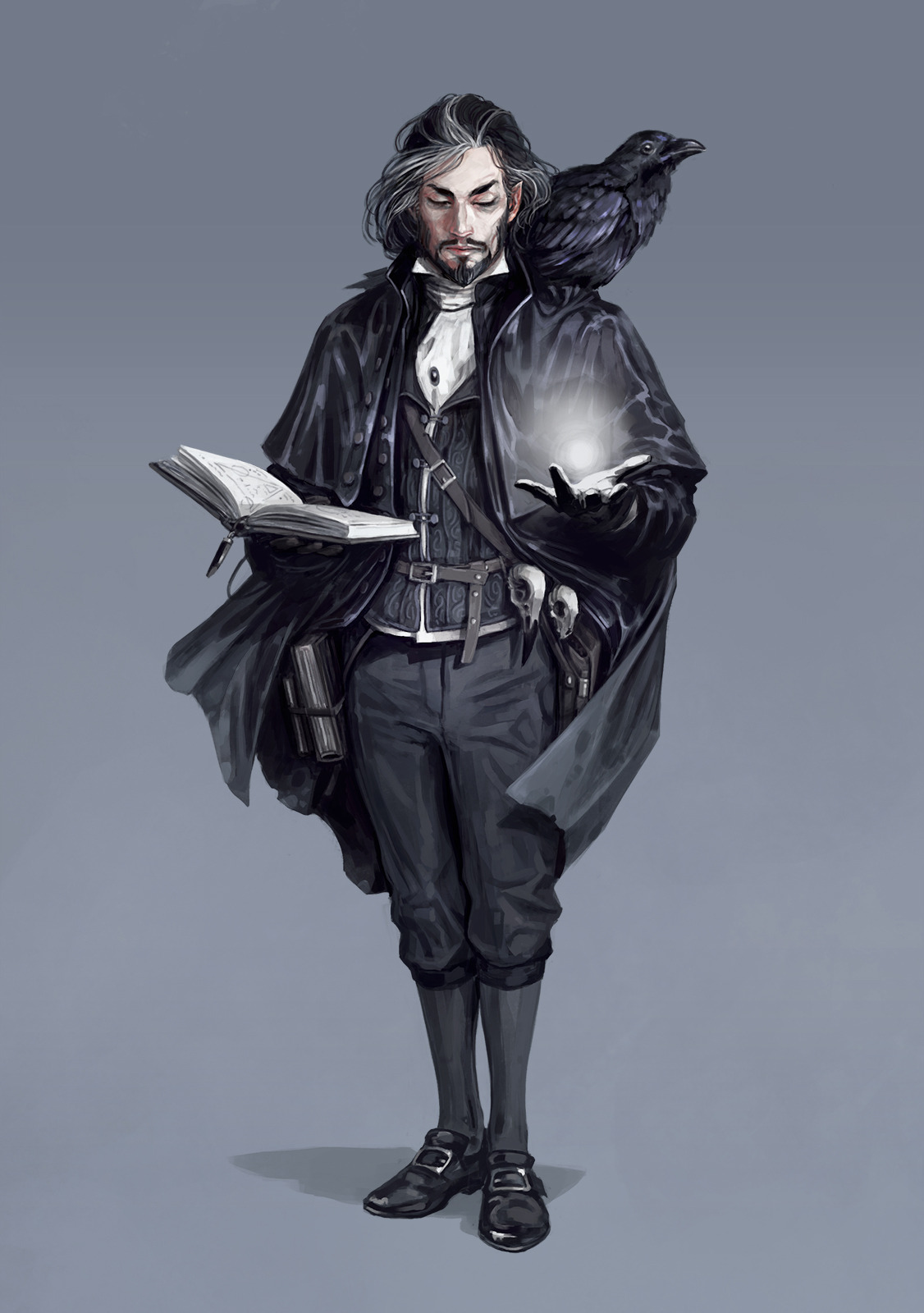The image depicts a man with long dark hair, a mustache, and a goatee, dressed entirely in black. He wears a black trench coat, black pants, knickers, long black boots, black socks, and a white shirt with black bands around it. The man is facing forward, and his white hair is interspersed with patches of black. Perched on his left shoulder is a black crow, gazing to the right. In his right hand, he holds an open book, which appears devoid of text, and in his left pocket, there are visible daggers. Additionally, there is a mystical white glow emanating upwards from his hand. The background is a simple, unembellished gray, underscoring the dark and enigmatic theme of the digitally created image.